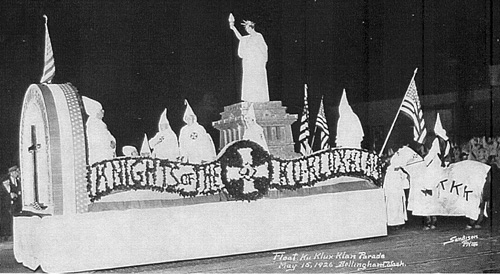The black-and-white photograph captures a disturbing scene from a Ku Klux Klan parade in 1926. Central to the image is a float mounted on a vehicle, prominently displaying the Statue of Liberty. The float is draped with numerous American flags, with the most visible ones placed to the right side and the middle. Men dressed in the infamous white robes and hoods of the Ku Klux Klan surround the float, their cone-shaped head coverings adding an eerie presence. A cross is prominently featured in the center of the float, while another cross is situated within an arched structure to the left. To the front of the float, the text "Knights of the Ku Klux Klan" is clearly legible, while the initials "KKK" appear on a banner further emphasizing the group's identity. At the bottom right of the image, faint text in a small white font and a barely visible signature mark the photograph. The sky appears dark, adding to the ominous atmosphere of this racially-charged event.